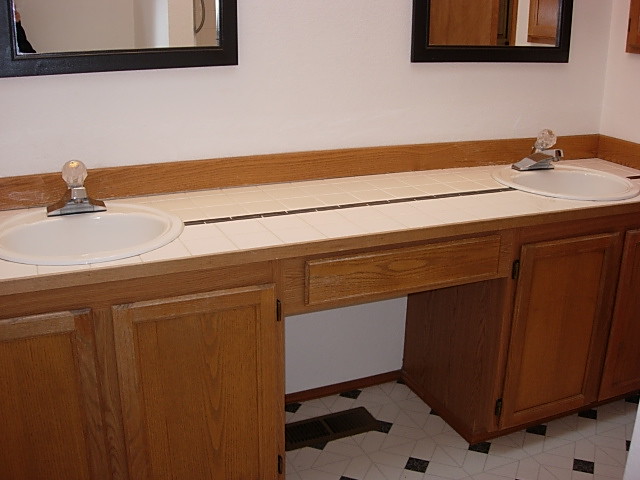This image captures the interior of a stylish bathroom featuring a double vanity set against a white wall. The vanity is crafted from a yellow pine cabinet, adding a warm, rustic charm to the space. Central to the vanity are two round, white sinks, each paired with a sleek, shiny chrome faucet and a single water control knob. Beneath each sink, the cabinet includes two yellow pine doors, offering storage, while a central drawer bridges the space between the sinks; below this drawer, an open area provides additional access and display space.

Both sinks are accompanied by mirrors edged in a sophisticated black frame, reflecting other parts of the bathroom and adding depth to the setting. The floor is adorned with a mostly white tile pattern, featuring small square tiles interspaced with black ones arranged in a diamond pattern, adding visual interest. In the open area underneath the vanity, a floor HVAC vent is visible, hinting at the room's functional elements.

The walls are painted a clean white, and in the upper right corner of the image, a partial view of what seems to be a medicine cabinet or another storage unit can be seen, though its details are not fully captured. A distinct black line of tiles runs across the vanity's surface, connecting the two sinks and adding a cohesive touch to the design.